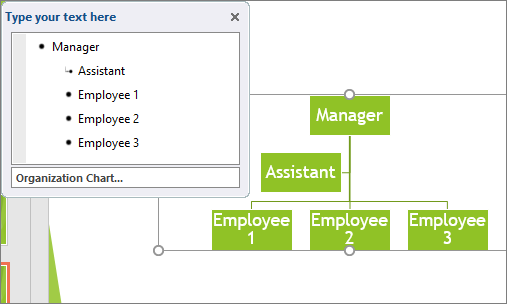The photo depicts an organizational chart with a hierarchical structure displayed on a mostly white background. Central to the image is a detailed chart starting from the top with a green-labeled "Manager" box. From the Manager, a line descends to connect with an "Assistant" box. Below the Assistant, three lines extend downwards connecting to "Employee 1," "Employee 2," and "Employee 3" boxes in sequence, forming a pyramid-like structure. The left side of the screen displays a text box labeled "Type your text here," allowing for customization of the names and details for each position. At the bottom, the chart is titled "Organization Chart." The bottom left of the image incorporates gray vertical lines adding subtle detail, while the overall background remains predominantly white. An 'X' symbol in the window hints at the diagram's editable nature.